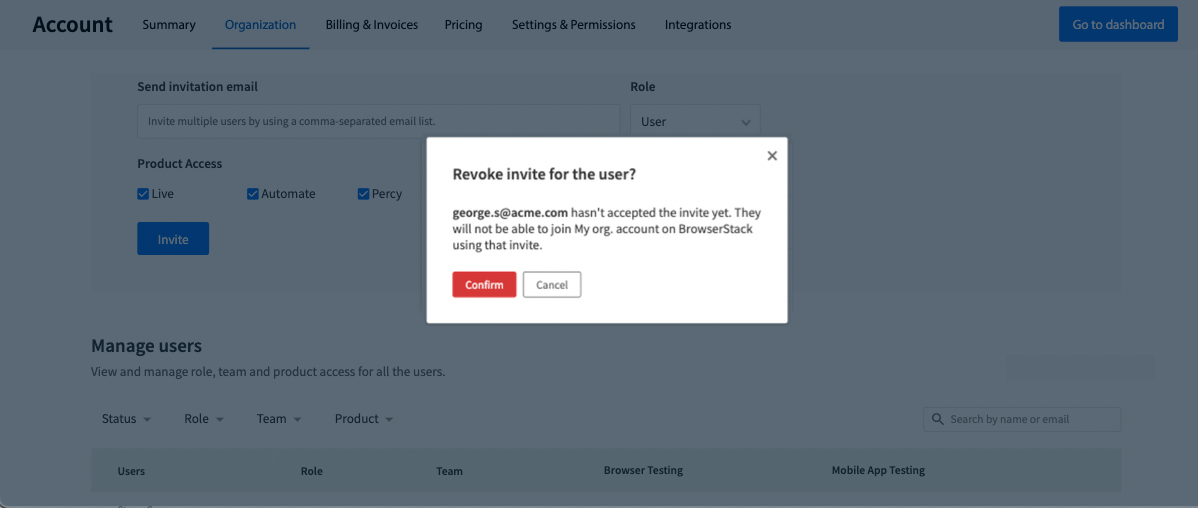The focal point of the image is a white square centered in the middle, displaying a message: "Revoke invite for the user?" Below this, it specifies that George (george@acme.com) has not yet accepted the invite to join the 'myorg.account' on the Slack browser. Two options are presented for the user: a red rectangular button labeled 'Confirm' and a white rectangular button labeled 'Cancel'. The background appears darker and less focused, emphasizing the importance of the central message. 

In the upper left corner of the image, the word "Account" is visible, followed by a vertical list of sections: "Summary," "Organization," "Billing and Invoices," "Pricing," "Settings and Permissions," and "Integrations." Toward the upper right corner, a blue box labeled "Go to Dashboard" stands out. Below it is an option to "Send Invitation Email," and a section detailing "Product Access" with "Live" and "Automate" both checked off in small blue boxes. Another section labeled "Manage Users" is also present. The overall composition places heavy emphasis on the invitation management, with peripheral elements providing additional context.